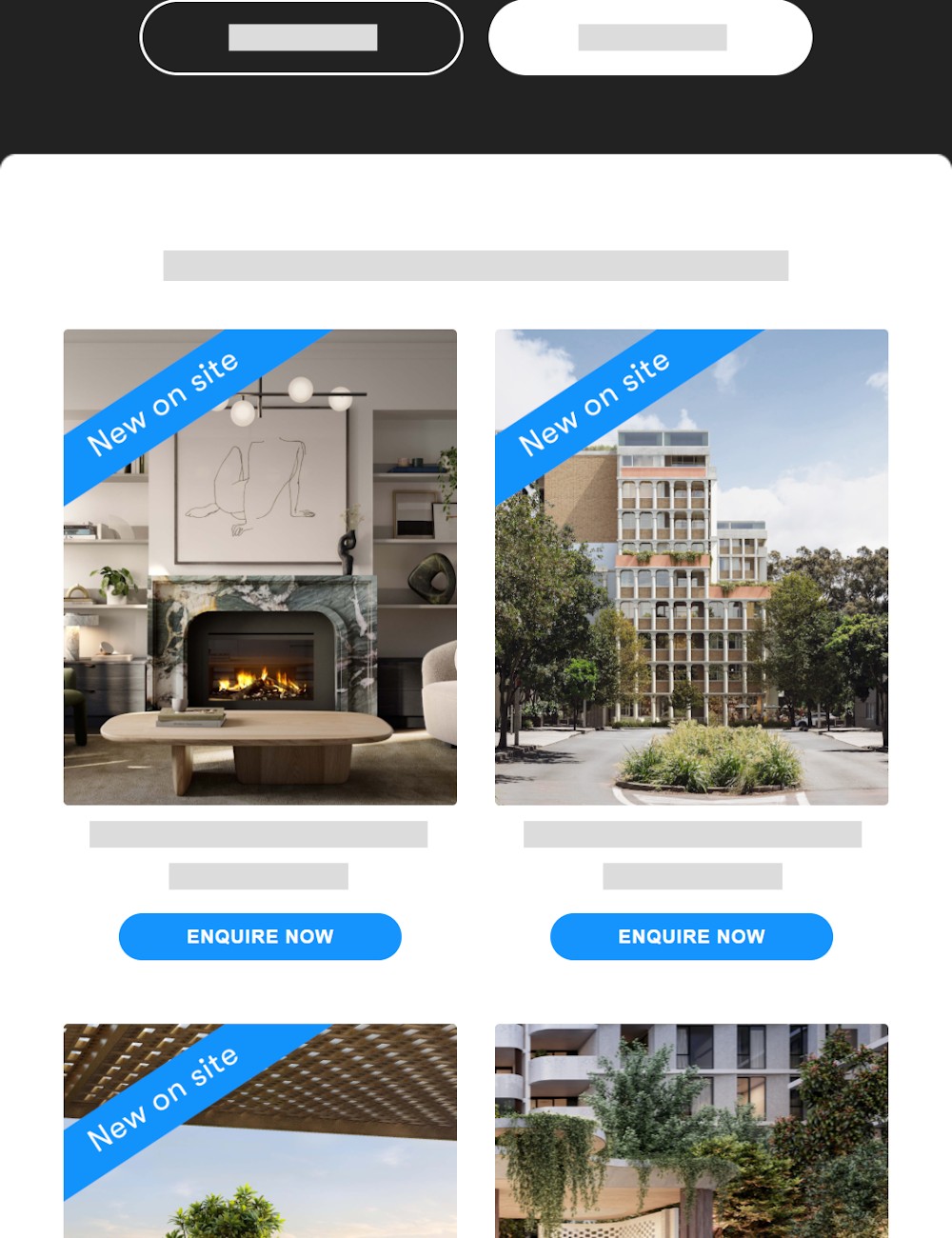Here is the cleaned-up and detailed caption:

---

A work-in-progress design for a template or website, showing an amateurish layout. The design features a prominent black header bar at the top, with two capsule-shaped elements—a black one on the left and a white one on the right—each containing a gray rectangle in the center. Below this header is a white panel with curved top corners, where the black header extends slightly down the sides.

Centered within the white panel is a gray field designated for text. Below this central area is a grid arrangement of four photographs, each representing different environments. The top left photo showcases the interior of an elegant house or apartment, featuring a marble fireplace and framed art above it. To the right of this is an exterior shot of a building with a courtyard that could double as a parking area, though its exact nature is unclear. 

The bottom left image appears to be an outdoor scene, possibly taken under a pergola, with a visible tree. The bottom right image displays the front of a building adorned with bushes and hanging vines over a rooftop or covered area. 

The top two photos and the bottom left photo have an angled blue banner labeled "NEW ON SITE" in large, obtrusively placed text, reflecting a poorly executed design choice. The bottom right photo is free of this banner. Below the top two photos are gray rectangles meant for text, with large blue capsule-shaped buttons labeled "Inquire Now." These buttons are missing from the bottom two photos due to the images being cut off.

---

This description provides a comprehensive and clearer picture of the design and its elements.